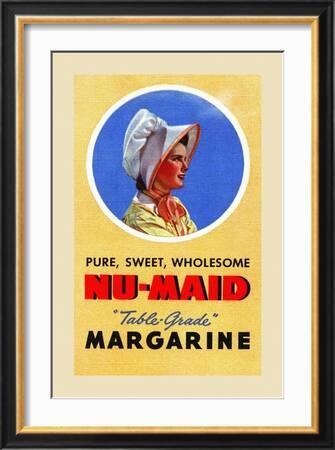This image showcases a framed, color advertisement illustration for table-grade margarine. The subject is a woman in a period costume, centered in the illustration and facing right in profile. She wears a Victorian-style white bonnet with a pink edge, a matching pink tie and bow under her chin, and has dark hair. Her light yellow dress features a white collar. The woman, who has a slight smile and looks slightly upward, is set against a blue background within a blue-rimmed circle. 

The text beneath her image is organized as follows: "Pure, sweet, wholesome" in black, followed by "NEW-MADE" in bold red, and "TABLE GRADE" in blue script within quotes. Below this, in all caps black text, is the word "MARGARINE." The entire illustration is framed, starting with a white mat, followed by a gold liner, and encased in a black outer frame. The overall style is reminiscent of old-fashioned advertisements, with its vintage charm accentuated by the portrait orientation and detailed period apparel of the featured woman.